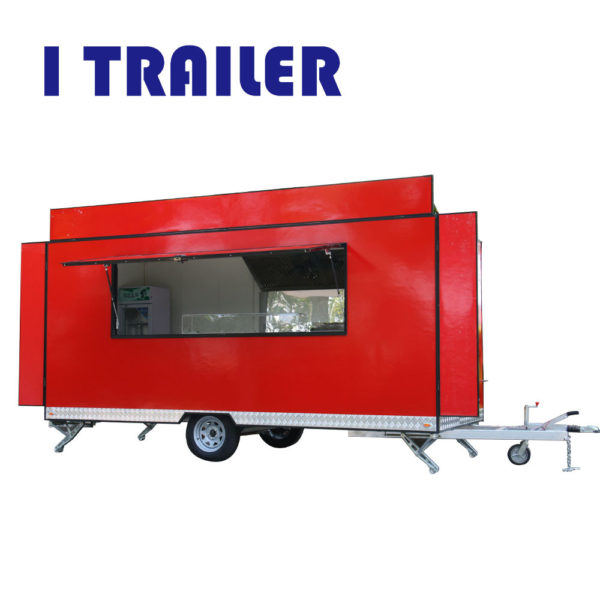The image displays a large, bright red trailer with a black trim that is reminiscent of a food truck. Positioned against a stark white background, the eye is initially drawn to the top left corner where the word "iTrailer" is emblazoned in bold, blue font. Dominating the majority of the image is the trailer itself, striking in its firetruck-red color. A notable feature is a large, rectangular window in the center, covered by a foldable awning that is also red, held up by silver hinges on either side. Below the main body of the trailer, there is a small silver metal trim running along the bottom edge, accompanied by a silver trailer hitch. The trailer rests on two rear tires with silver rims and also includes a small, height-adjustable front tire near the towing attachment point. Inside the trailer, visible through the open window, is a pink refrigerator or freezer, suggesting its potential use as a food service vehicle.